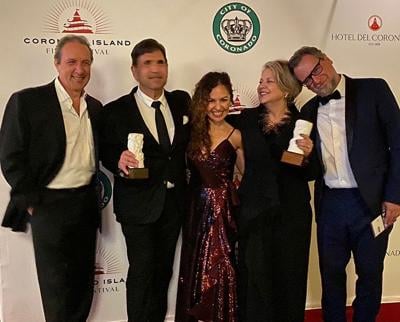In the image, five adults are standing in front of a detailed poster with the backdrop featuring a red mountain encircled by a white ribbon. Below this graphic, the text reads "City of Coronado" and "Hotel del Coronado." The poster background also reveals partial text hinting at "Coronado Island." In the center, there is a crown with a green circle surrounding it.

The group consists of three men and two women, all dressed in formal attire. The first man on the left is in a black suit and white collared shirt without a tie. The second man, standing next to him, also wears a black suit but pairs it with a white shirt and a black tie. The third man, situated on the right, is distinguishable by his black bow tie, glasses, and beard, complementing his black suit and white shirt.

Between the men, the two women display contrasting styles. The woman in the center is adorned in a maroon strap dress with a floral print, while the woman beside her opts for an elegant all-black skirt suit. The formal setting suggests they are attending a red carpet or ceremonial event.